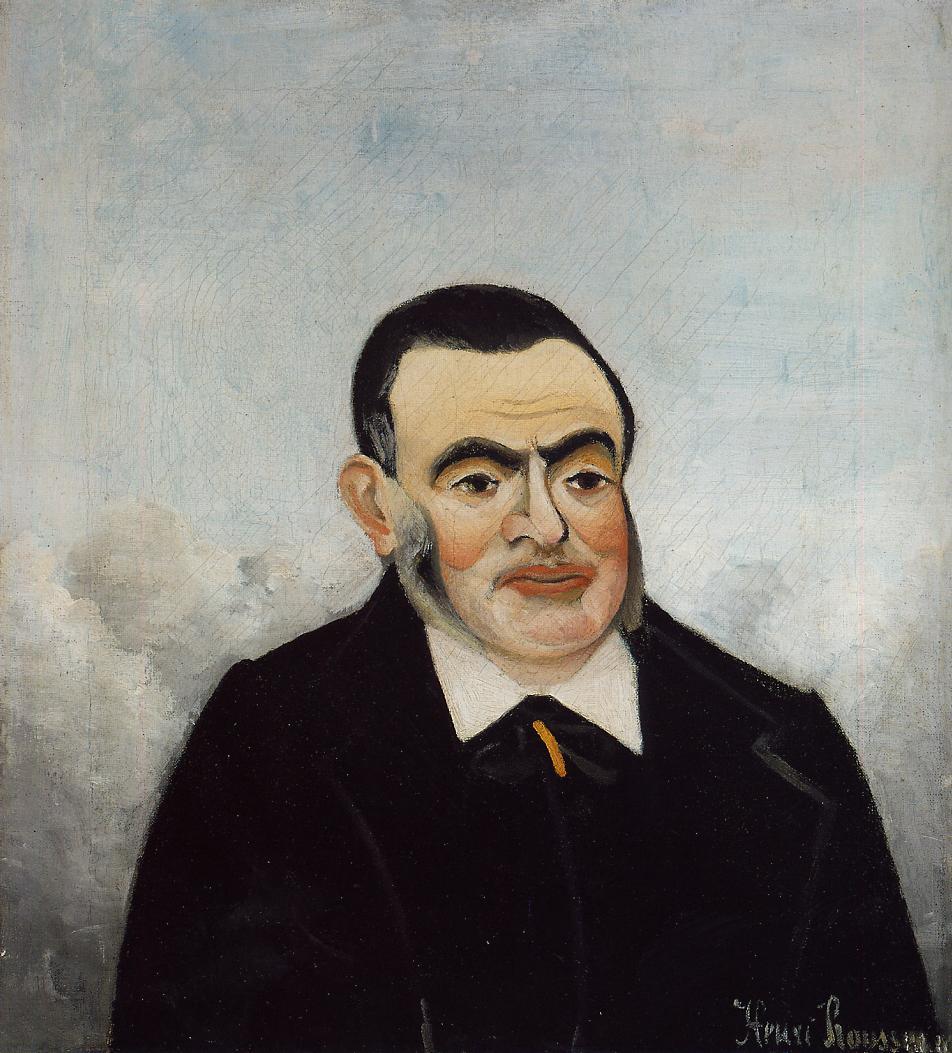The image is an oil-on-canvas painting of an older, middle-aged man set against a cloudy gray background. The man is slightly overweight and is depicted sitting and looking slightly away from the viewer, capturing a vintage and contemplative demeanor. He has short black hair with gray mutton chops and a bushy black unibrow. His facial features include small eyes, a large crooked nose, and thick pinkish-red lips. He is dressed in a black outfit with a white collared shirt underneath, and an additional green velvety garment. A black jacket with an orange line, likely part of a tie or scarf, adds to his distinguished appearance. The artist's signature, which is hard to read but appears to start with "Henri" or "Henry," is located in the bottom right corner. The painting's striking use of contrasts and detailed brushwork makes it a noteworthy piece that could be found in a museum.